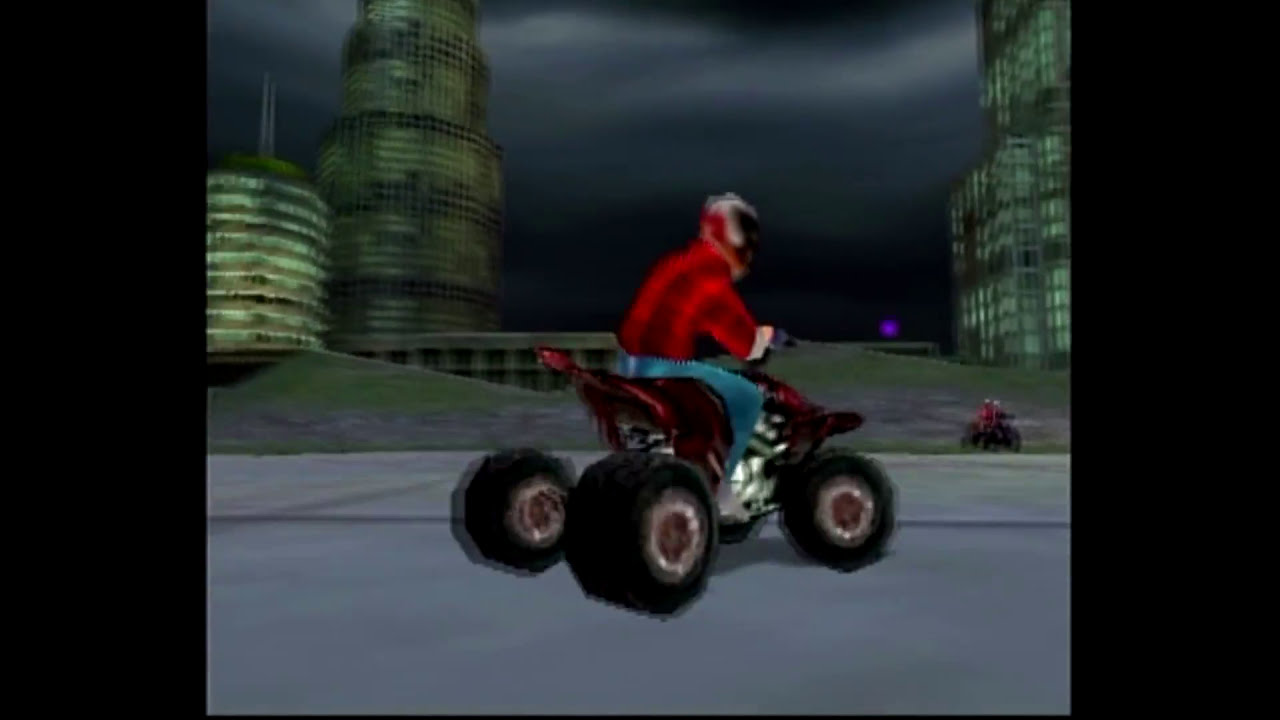The image appears to be a still from a video game, reminiscent of older consoles like the Nintendo 64, PlayStation 2, or Sega Dreamcast. It features a side view of a man riding an ATV on a concrete path. The man is wearing a distinctive red long-sleeve shirt with a plaid pattern, blue jeans, and a white and red helmet. The ATV he rides is predominantly maroon with large black tires, the back tires being bigger than the front ones.

The setting includes two structures on the left side: a tall, cylindrical tower with greenish windows and another shorter building also exhibiting green hues and numerous windows. On the right side, there is a blurry, similarly greenish building. The grass, vividly green, stretches ahead of the man, intermixed with flat gray stones. The sky overhead is a dark, ominous gray, suggesting stormy or rainy weather, adding to the dramatic ambiance of the scene. No other people are visible, and the man's face is somewhat blurred, indicating motion or the video game's graphical limitations.